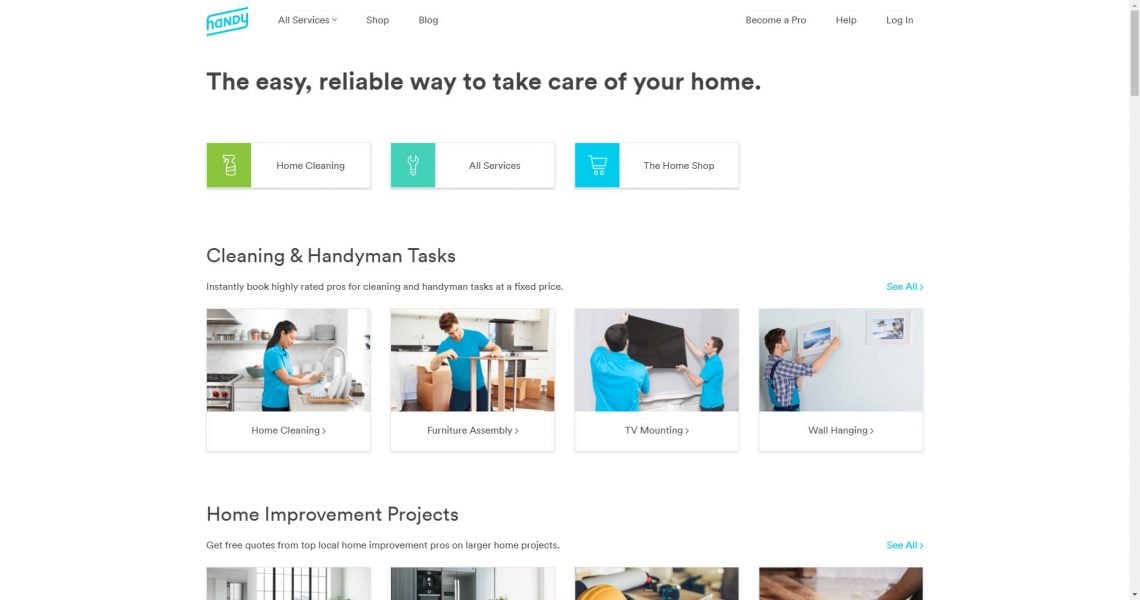The landing page for the Handy website is well-organized and designed to be user-friendly. Located in the upper left-hand corner is the Handy logo. Adjacent to it are navigation options including "All Services," "Shop," and "Blog." On the far right-hand side of the top menu, users will find links to "Become a Pro," "Help," and "Log In."

Dominating the central area of the page is the main headline: "The Easy, Reliable Way to Take Care of Your Home." Below this, three prominently displayed buttons offer pathways to specific services: "Home Cleaning," "All Services," and "Home Shop."

Further down, there's a section dedicated to "Cleaning and Handyman Tasks," with a subheading that promises, "Instantly Book Highly Rated Pros for Cleaning and Handyman Tasks at a Fixed Price." Four images illustrate various services, showcasing professionals in blue shirts working in suburban home environments. The services depicted are: 
1. **Home Cleaning**
2. **Furniture Assembly**
3. **TV Mounting**
4. **Wall Hanging**

Each image features one or two professionals in blue shirts actively engaged in their respective tasks. 

Beneath this section, there is another category labeled "Home Improvement Projects." Although the images here are partially cut off and do not clearly reveal all details, it is evident there are four categories. Accompanying text states, "Get Free Quotes from Top Local Home Improvement Pros on Larger Home Projects," inviting users to explore comprehensive home improvement services.